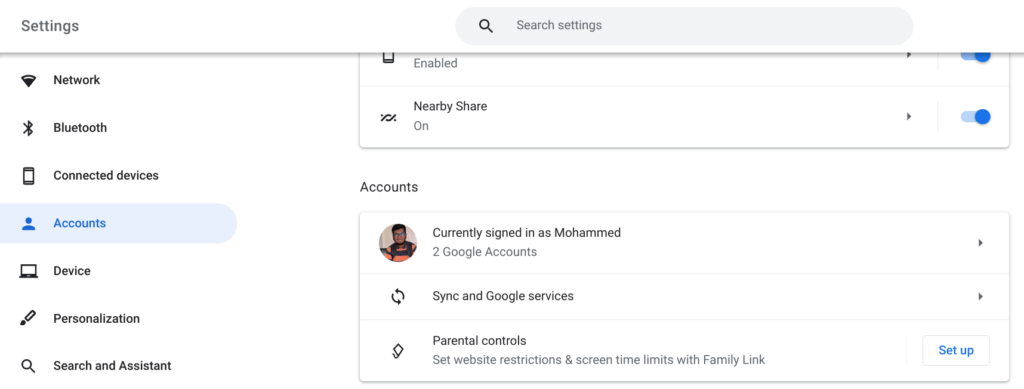The image depicts a computer screen displaying a detailed Settings page. On the right side of the screen, a prominent search box with a gray background is visible under the "Search Settings" area. As you scan further down, the following sections are listed sequentially: "Network," "Bluetooth," "Connected Devices," "Accounts," "Device," "Personalization," and at the bottom, "Search and Assistant."

In the upper part of the screen, there are notable sections labeled "Enabled" and "Nearby Share," both of which are turned on. Further down, within the "Accounts" section, there is a profile picture showing a person inside a circle. Below this icon, it indicates the user is currently signed in as Mohammed, with two linked Google accounts. Additional settings within this section include "Sync and Google Services" and "Parental Controls."